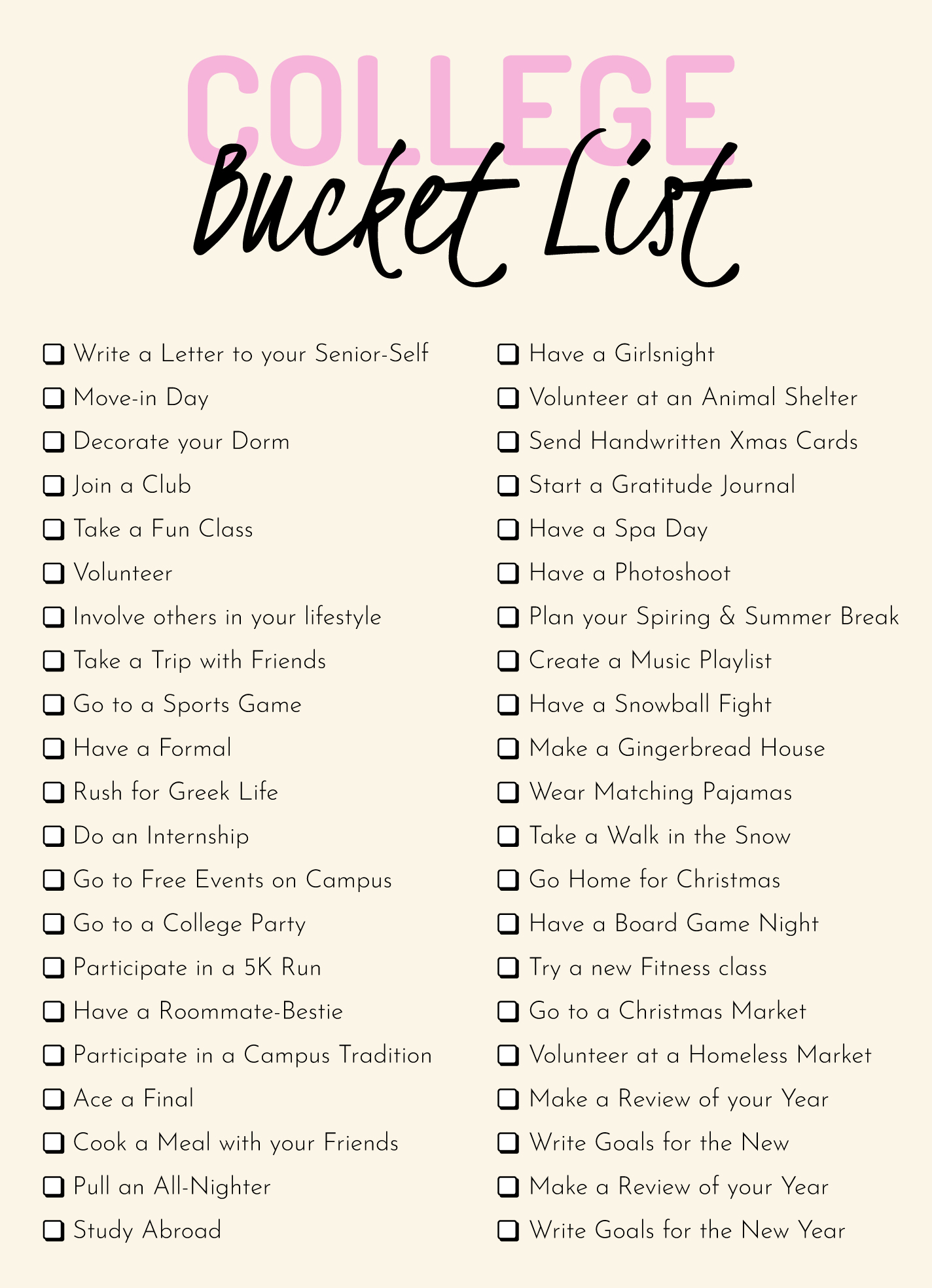The image depicts a detailed "College Bucket List," designed against a beige background reminiscent of something you might find on Pinterest. The title "College Bucket List" features "College" in pink, bold letters and "Bucket List" in a cursive, curly black font. Below the title, there is an extensive, unchecked checklist with about 40 different items spanning two columns. Each item on the list has a checkbox next to it for ticking off completed tasks. 

In the left column, the list includes activities such as "write a letter to your senior self," "move in day," "decorate your dorm," "join a club," "take a fun class," "volunteer," "involve others in your lifestyle," "take a trip with friends," "go to a sports game," "have a formal," "rush for Greek life," "do an internship," "go to free events on campus," "go to a college party," "participate in a 5K run," "have a roommate bestie," "participate in a campus tradition," "ace a final," "cook a meal with your friends," and "pull an all-nighter."

In the right column, the activities listed are "study abroad," "have a girls' night," "volunteer at an animal shelter," "send handwritten Christmas cards," "start a gratitude journal," "have a spa day," "have a photo shoot," "plan your spring and summer break," "create a music playlist," "have a snowball fight," "make a gingerbread house," "wear matching pajamas," "take a walk in the snow," "go home for Christmas," "have a board game night," "try a new fitness class," "go to a Christmas market," "volunteer at a homeless shelter," "make a review of your year," and "write goals for the new year."

This visually appealing checklist aims to guide students through a fulfilling college experience, blending academic achievements with personal and social milestones.